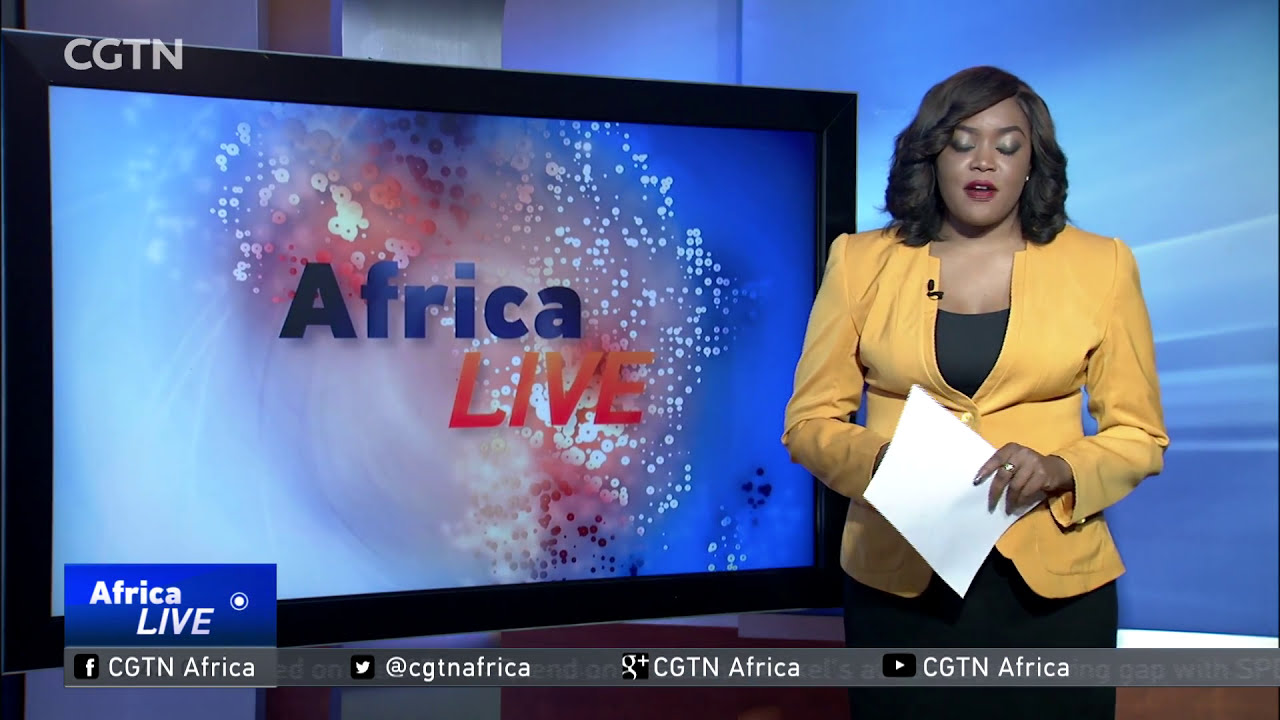The image is a still frame from a CGTN news broadcast featuring a black woman newscaster positioned on the right side. She's wearing a yellow blazer buttoned below her chest, over a black shirt, and a black skirt. Her long black hair frames her face, and her eyes are closed with her mouth slightly parted, as if she is speaking. She wears a ring on her left finger and is holding a sheet of paper. To the right, behind her, a large flat-screen TV with a black frame displays the text "AFRICA LIVE" in blue and red fonts against a swirling blue and red backdrop. The top left of the image features a grey "CGTN" watermark. The bottom left corner shows a blue box with "AFRICA LIVE" in white font and social media icons for Facebook, Twitter, Google Plus, and YouTube.